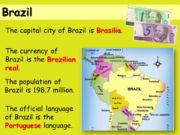This image is a detailed screenshot taken from a computer screen. The main section features a square with a green background. At the top of the square, there's a horizontal yellow line that is labeled "Brazil" on the left side in black text. 

To the right of this line, two currency bills are illustrated; one is green and the other is purple, suggesting they are representations of Brazilian currency. 

The content within the green background provides various pieces of information about Brazil. The first line states "The capital city of Brazil is Brasília," where "Brasília" is highlighted in red. The second line reads, "The currency of Brazil is the Brazilian Real," with "Brazilian Real" also emphasized in red. Following this, the text indicates that the population of Brazil is 198.7 million. The final line on the bottom left mentions, "The official language of Brazil is Portuguese," with "Portuguese" in red.

Additionally, the bottom right corner of the square contains a small map of Brazil. This map depicts Brazil in yellow, with surrounding land and bodies of water on the left and right sides, respectively.